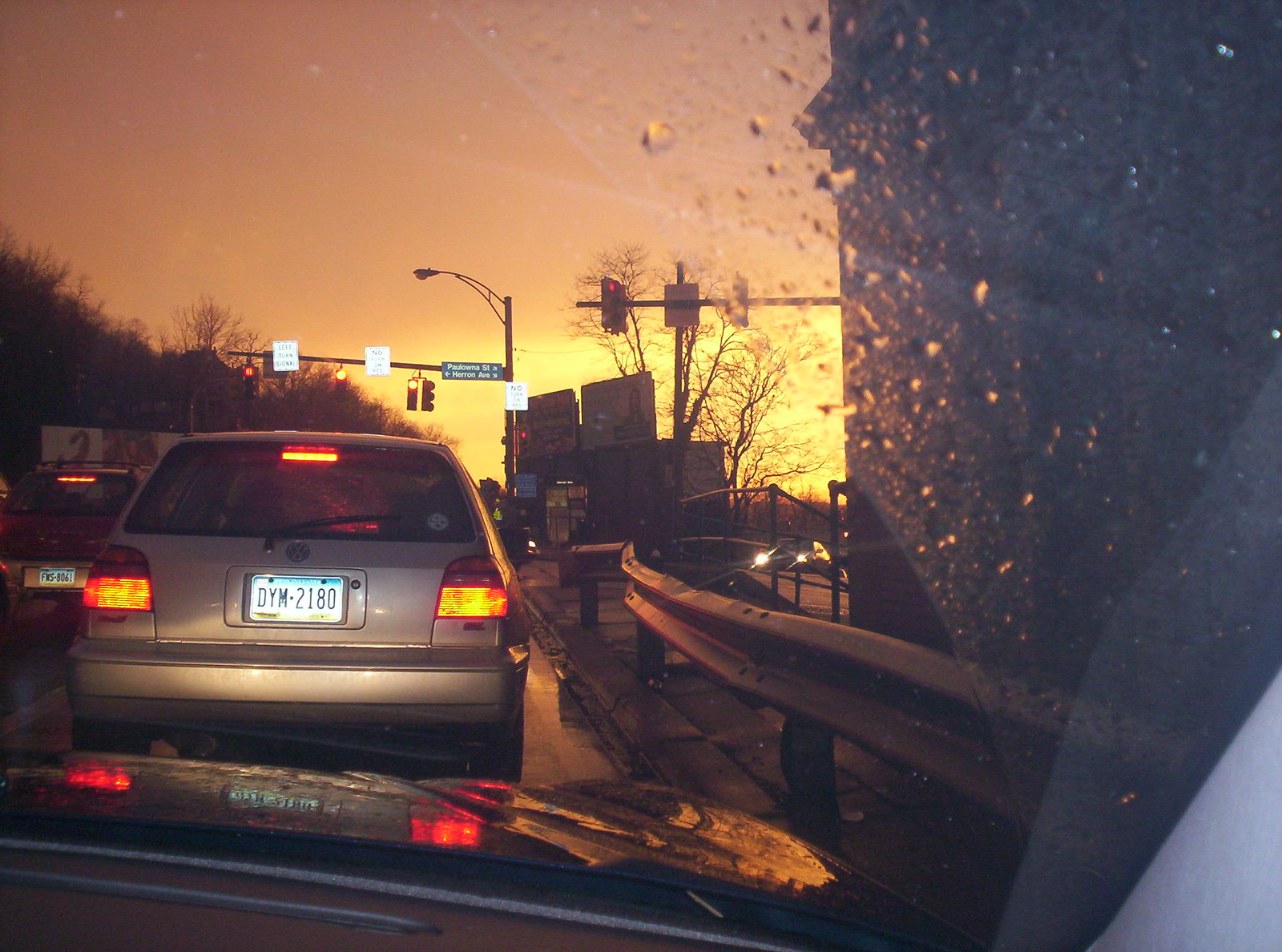This image captures a scene from inside a car, taken either early in the morning or late at night. The sky is adorned with a beautiful orange-peach hue, lending a serene atmosphere to the photograph. On the right side of the frame, a guardrail runs alongside the road. Directly ahead, a silver Volkswagen sedan with a white license plate bearing the dark letters "DYM-2180" sits stationary at an intersection, its brake lights glowing red. Above, a streetlight casts its illumination, flanked by two red traffic lights and a green street sign that is indistinct. In the distance, a taller streetlight provides additional lighting to the scene.